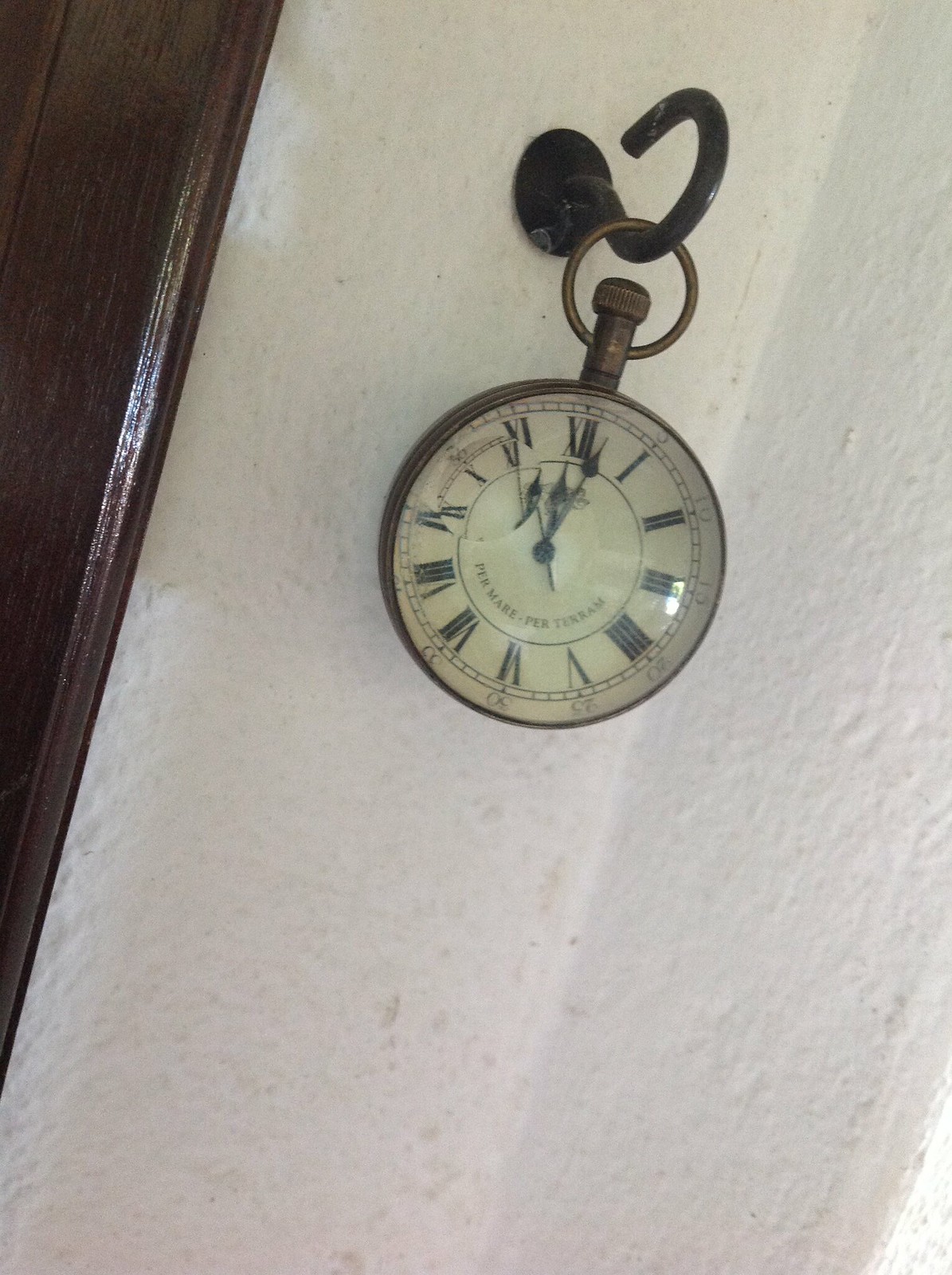The image features a large antique pocket watch, styled to resemble a traditional grandfather clock, hanging from a decorative wall hook typically used for planters. The pocket watch, which may either be an oversized functional clock or an actual pocket watch presented in a highly magnified view, prominently displays Roman numerals. It appears to be showing a time slightly past 12:00. The background is predominantly white, possibly indicating a plain wall or an indistinct surface, with a hint of wood visible, suggesting a rustic or vintage setting. Due to the close-up nature of the photograph, the precise dimensions of the clock remain unclear, adding an element of intrigue to its historical charm.